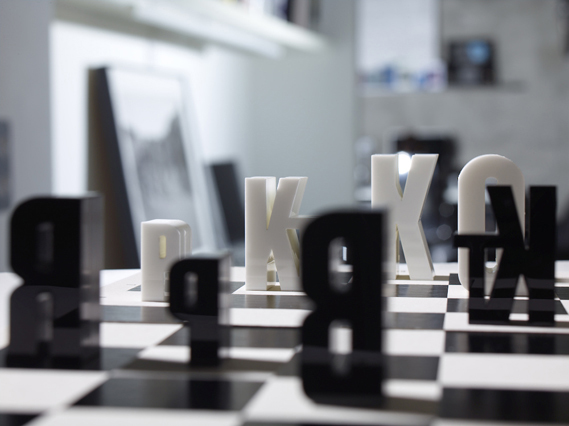A detailed color photograph captures an unconventional chessboard scene. The chessboard features a classic black and white checkered surface, with chess pieces uniquely shaped as letters. In this artistic setup, the letters represent the first initial of traditional chess pieces: a white 'K' for King, another white 'K' for King or Knight, and an 'O' which could represent the Queen or just be part of the thematic decor. Surrounding them are several black pieces, including a 'P' for Pawn, a reversed 'B' for Bishop, a smaller 'K' for King or Knight, a 'KT' for Knight, and a reversed large 'R' for Rook. The pieces are scattered across the board, creating a playful yet sophisticated look. Behind the chessboard, a warmly lit, blurry interior scene reveals white and gray walls adorned with indistinct picture frames. A black shelf with a square object sits close to the wall, adding depth to the cozy domestic setting that captures a casual yet intriguing chess game in progress.